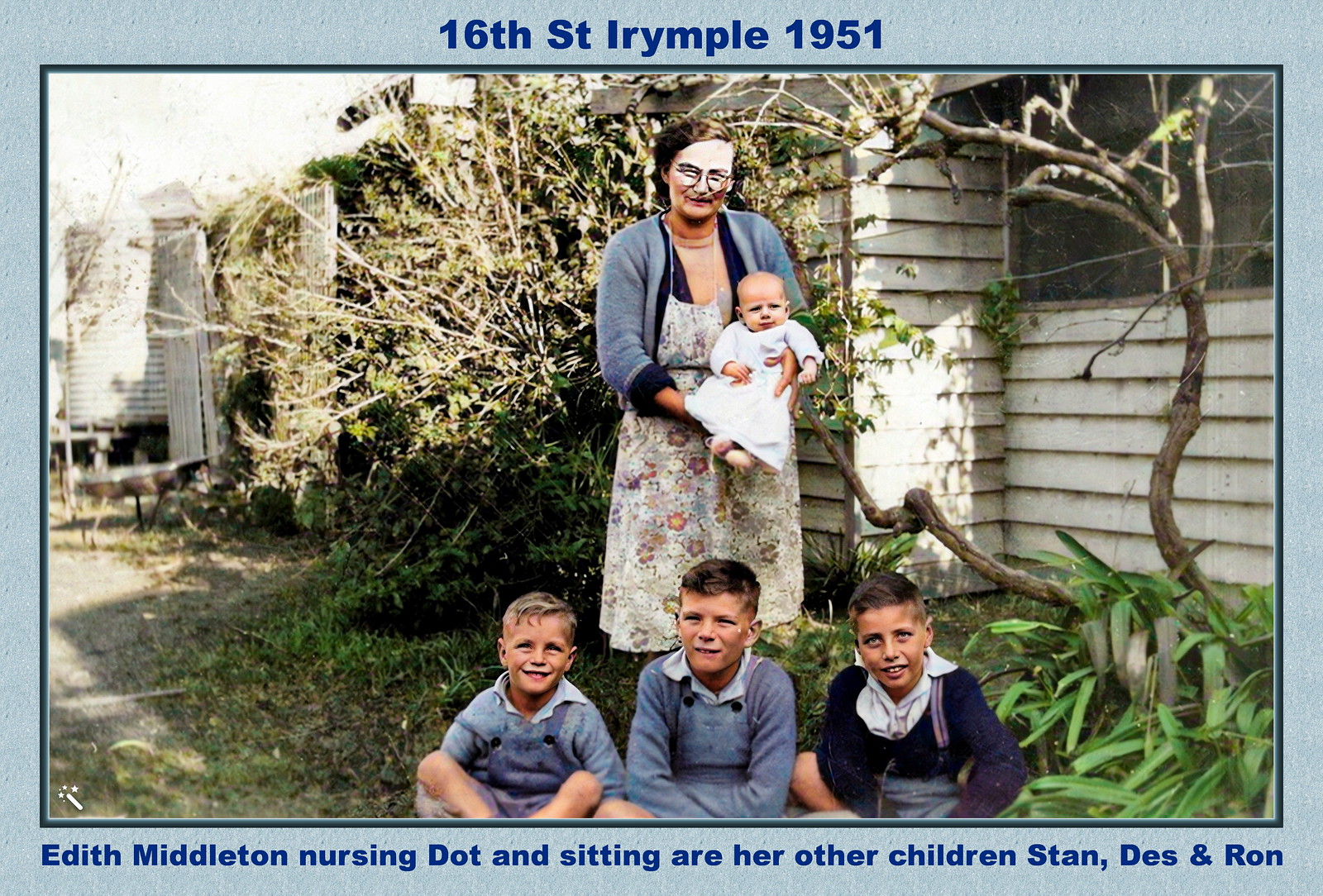This detailed color daylight photograph captured in 1951 features a woman identified as Edith Middleton holding a baby named Dot, with her three other children—Stan, Des, and Ron—sitting on the ground in front of her. The image is set within a light blue digital frame with dark blue text both at the top and bottom. The top text reads "16th Street, Irymple, 1951," while the bottom states "Edith Middleton Nursing Dot, and sitting are her other children, Stan, Des, and Ron."

The background reveals a wooden building extending down the block, potentially accompanied by some metallic silos. Surrounding the building are both green and quite possibly dead or autumnal trees. The scene also includes some smaller bushes and greenery.

The boys, all donning blue attire, sit closely together. The youngest, on the left, is dressed in blue overalls and a blue shirt, his light hair slicked to the side with a bright smile on his face. The middle boy, less cheerful and dark-haired, wears a blue shirt, while the eldest on the right, also with dark hair, sports a dark blue top and suspenders. The mother, standing behind them, has fair skin, brown hair, and glasses. She wears a blue sweater over a white-flowered dress, and holds the baby, Dot, who is clothed in a white dress. The setting appears to be outdoors in front of a white-sided house, adding a homely and nostalgic touch to the family snapshot.